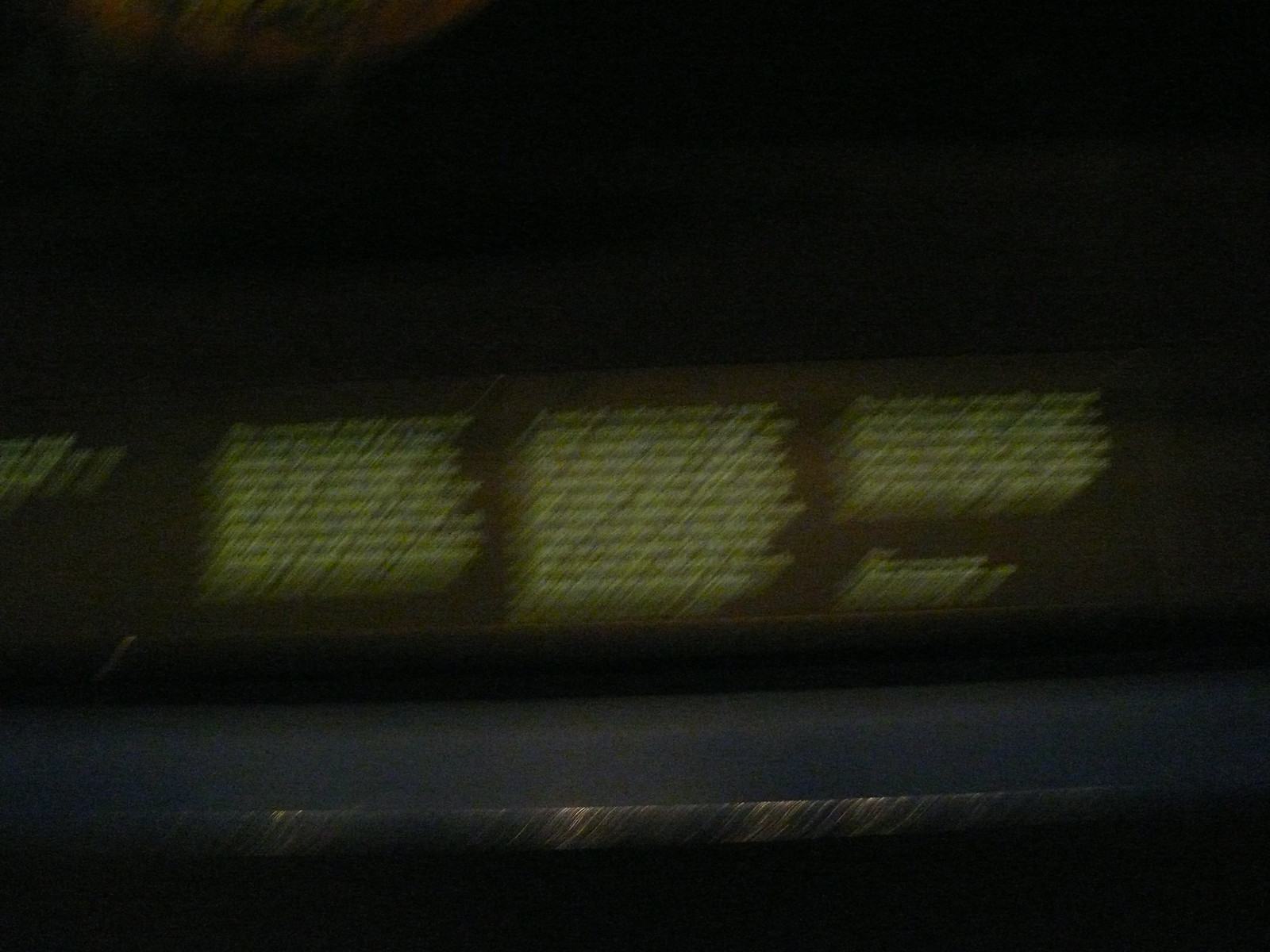The photograph is in color but appears predominantly blurred, lending it a somewhat abstract quality. The background is uniformly dark, especially towards the top left corner. Here, a half-circle with a gradient brownish-orange hue emerges, gradually lightening as it descends down the image.

In the middle of the photograph, a blurry band appears, marked with irregular sections of yellow and white, resembling a dashboard with indistinct buttons. The edges of these buttons, particularly on the right, are not clearly defined.

As the image continues downward, the colors transition into darker tones, including a dark gray section. This darker palette culminates at the bottom of the photograph, which is almost entirely black.